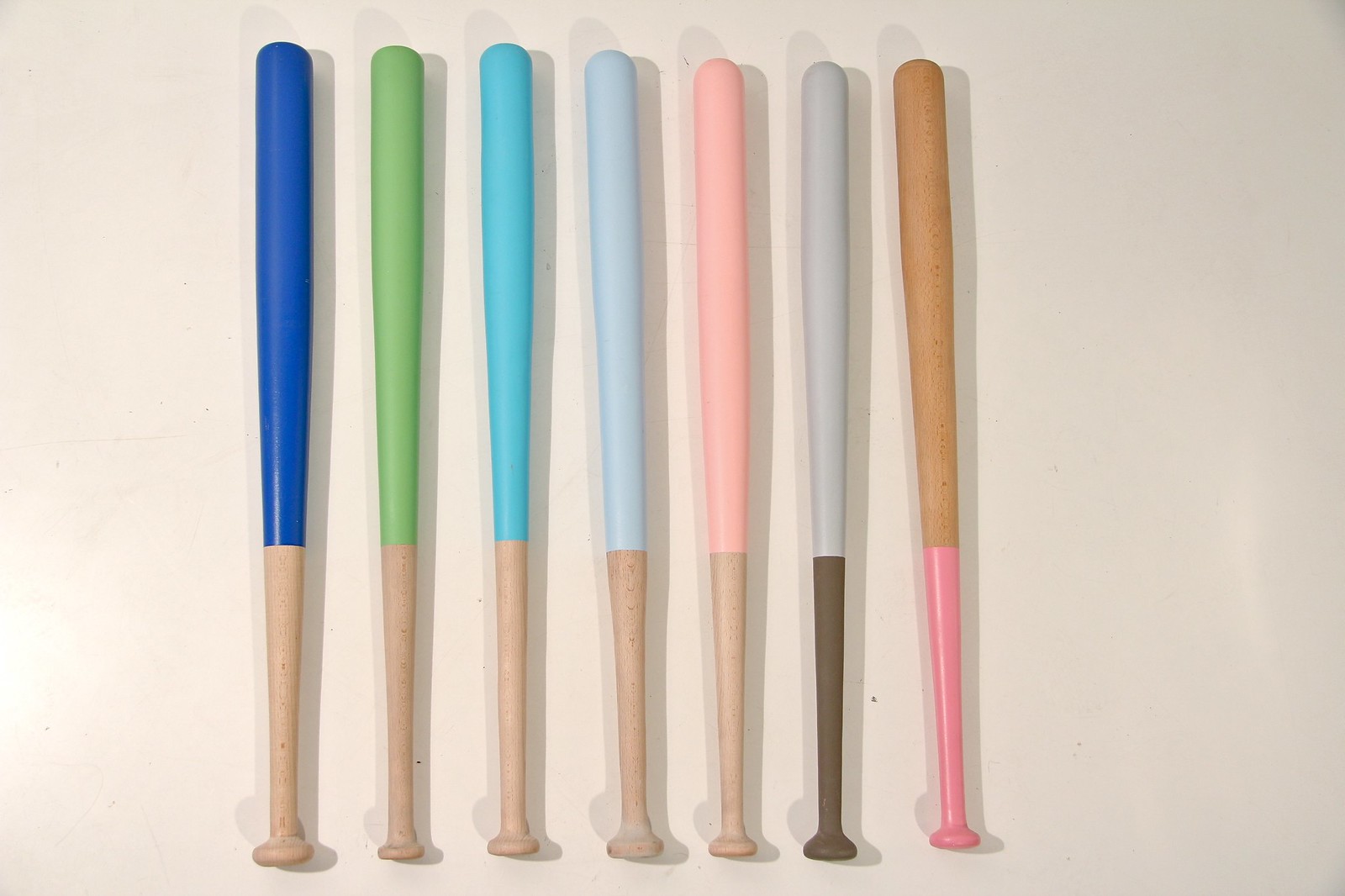This image features seven vertically aligned baseball bats set against a beige background. Despite its photorealistic appearance, there’s an artificial feel to it, likely because the bases of the three leftmost bats appear warped or twisted. Each bat has a distinctively colored top: starting from the left, the colors are blue, light green, bright blue, very light purple/blue, light pink, gray, and beige/wooden. The bats' handles mostly share a common light wooden color except for the last two to the right; one has a dark wooden handle, and the other has a pink wooden handle. The image blends a realistic style with noticeable digital manipulations, particularly in the inconsistencies at the bottoms of the bats.